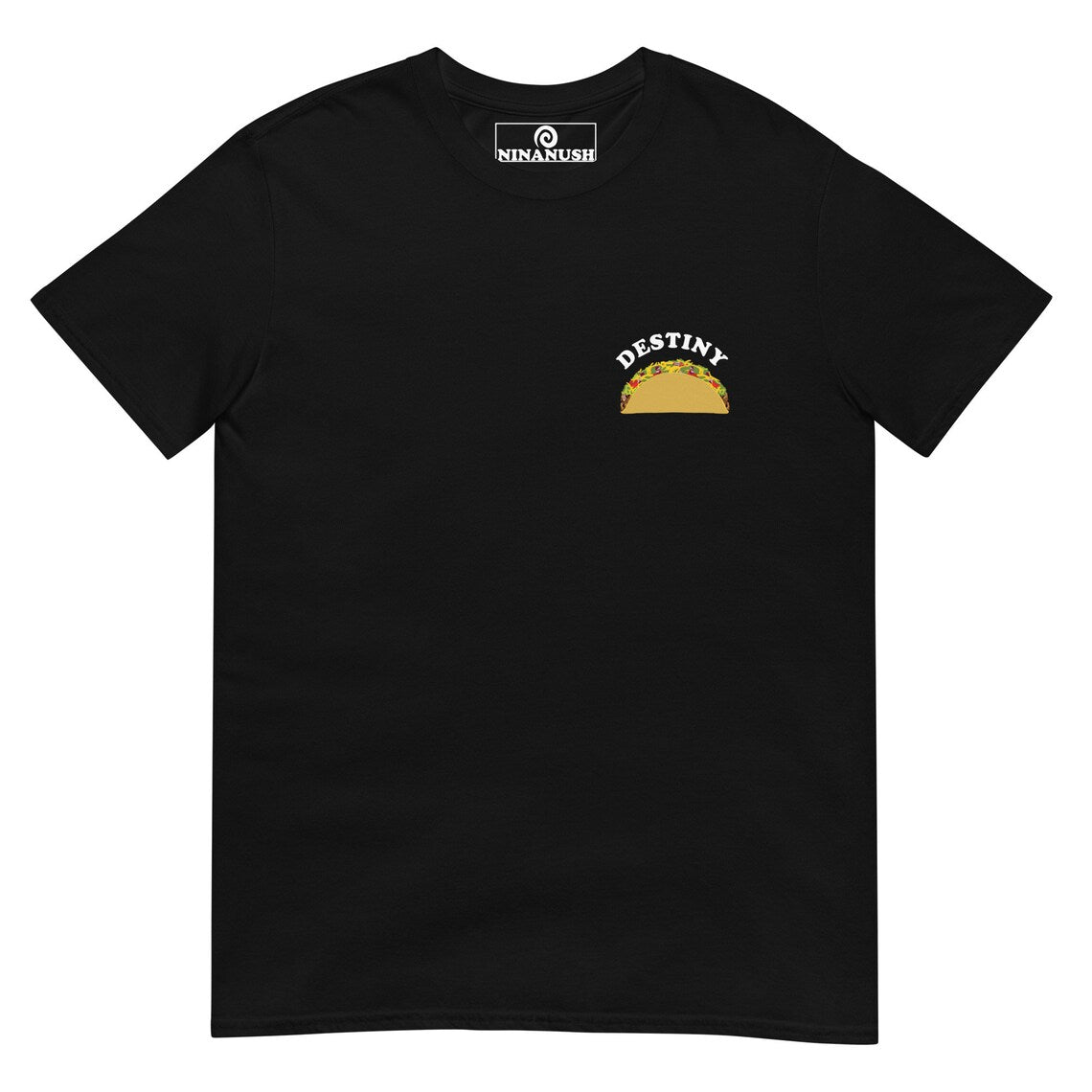This is a clear, high-resolution photograph of a black, freshly laundered and ironed crewneck t-shirt, isolated against a plain white background. The t-shirt features a printed label at the back of the neck with a white border, displaying a swirled graphic logo and the text "NINANUSH" in all capital letters. In the top right-hand corner of the chest area, approximately where a pocket would be, there is a detailed graphic that includes the word "DESTINY" arched in white, uppercase letters above an illustration of a taco with a tan shell, filled with vibrant ingredients like light green lettuce, red tomatoes, yellow cheese, and meat. The image is in sharp focus, showcasing the precise details of the t-shirt's design elements.